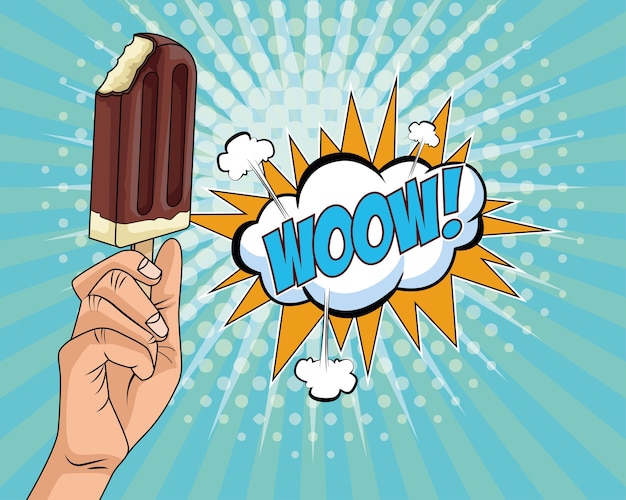The image is a vibrant, cartoony illustration of a chocolate-covered ice cream bar, prominently placed at the top left corner of a square frame. The ice cream bar, with a bite taken out of it, reveals creamy white vanilla ice cream inside, while the bottom part of the bar remains uncovered showcasing its vanilla center. The bar is attached to a brown stick held by a hand that emerges from the bottom of the image. The hand is depicted in a pinkish hue, enhancing the comic style.

In the middle of the image, the word "WOW!" is presented in playful blue letters, stylized as W-O-O-W with an exclamation mark. This text is set within a fluffy white cloud, which is layered on top of a striking orange starburst shape. The background features alternating radiating spokes in light green and light blue, adding a dynamic sense of movement and excitement. Overlaying this background are patterned white dots reminiscent of comic book art, and a translucent white starburst further accentuates the central "WOW!" message. The vivid colors and minimal shading contribute to the image's overall two-dimensional, playful, and eye-catching aesthetic, making it resemble an advertisement for a delightful, irresistible treat.